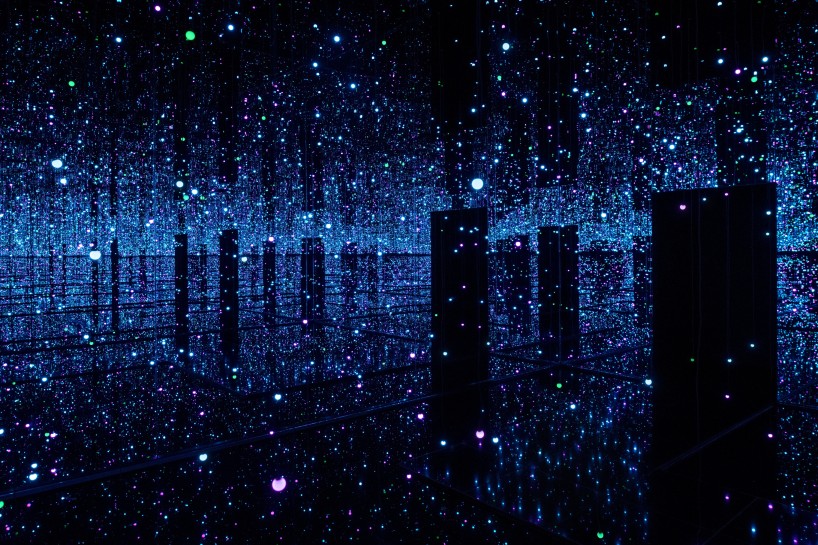This image portrays a mesmerizing night scene that can be interpreted as either an urban cityscape or an abstract, futuristic landscape. Primarily, the image is shrouded in darkness, with the background almost entirely black. It is dotted with an array of white lights and speckles of varying sizes, some large and vivid, others small and faint. These glowing points create an impression similar to falling snow, shimmering confetti, or vibrant disco lights.

In the center of this scene, tall, rectangular, and square-shaped objects are scattered, reminiscent of imposing skyscrapers. These structures spaced apart, contribute to a sense of a monolithic skyline, which could be viewed as buildings along a waterfront or a scene straight out of a high-concept sci-fi film like The Matrix. The congregated white speckles around these structures give off a faint light blue hue, intensifying the ethereal quality of the scene. This interplay of lights and darks creates a hypnotic view, suggesting a vast field of tiny lights or a special effects shot for a laser display.

Overall, this dense constellation of lights against a deep black background fosters an atmosphere of both a bustling nocturnal city and a surreal, otherworldly environment.